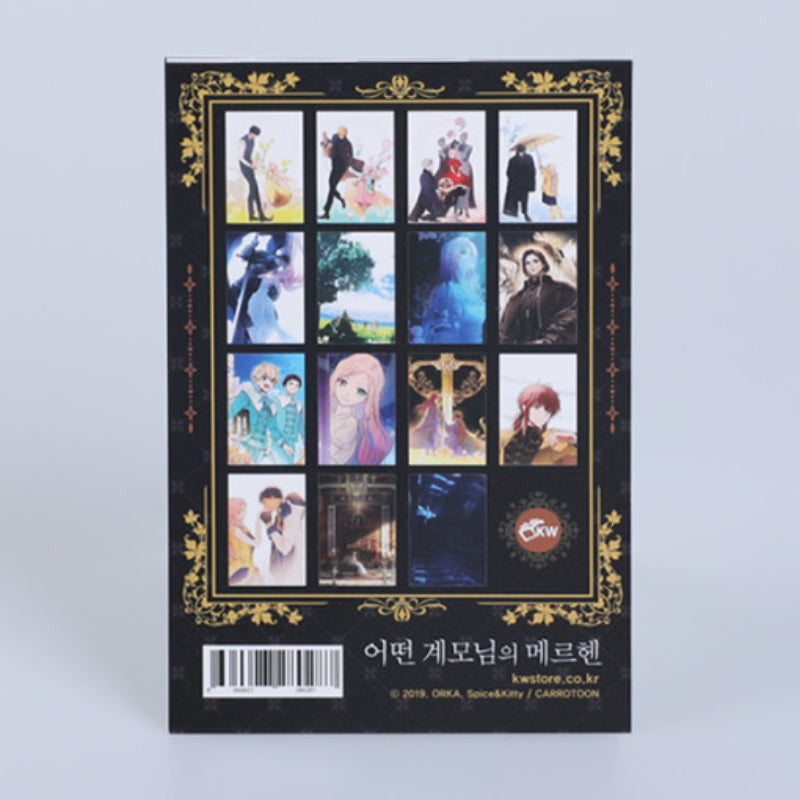The image displays a collection of pictures or cards, seemingly related to various Disney films, each featuring distinct Disney characters within individual squares. These character images are set against a backdrop that resembles a black picture frame with intricate gold designs. At the bottom of the image, there is text in a non-English language, alongside the website "kwstore.co.kr" and a copyright note from 2019. A barcode is also visible in the bottom left corner of the image.